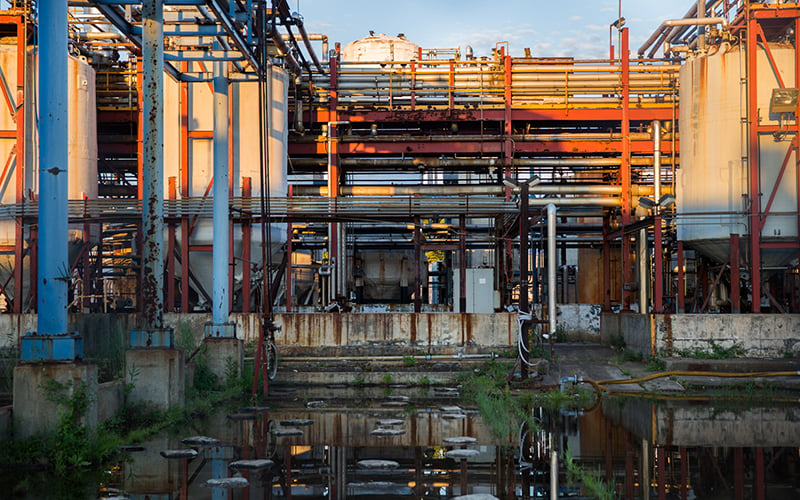The image captures an outdoor abandoned industrial plant, reminiscent of something out of Chernobyl, with complex and weathered machinery. Dominating the scene are numerous pipes and towering structures, including three large metal posts on the right and three white metal containers likely meant for storing substances. The left side of the image features three blue steel pillars supporting an overhead walkway. The plant is in disrepair, with broken pieces of metal and plastic in blue and steel gray hues scattered about. Red tubing snakes up and across the buildings amidst a tangle of interconnected pipes. The ground below reveals a wet, possibly flooded area, reflecting the machinery above, and scattered grass patches indicate prolonged neglect. The sky is bright, suggesting a sunny day, as its light highlights the varied colors of the machinery—blue, orange, white, and copper. Cement barricades in the distance add to the sense of industrial abandonment.